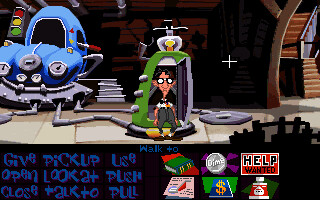The image appears to be a screenshot from a video game. On the left side, there is a whimsical, blue automobile with a cartoonish design, featuring a rounded shape and a front that resembles a mouth. Adjacent to the car is a traffic signal displaying the standard green, yellow, and red lights.

Additionally, a quirky character, presumably a man, is present in the scene. He is wearing amusing glasses with opaque white lenses, concealing his eyes. This character appears to be either seated inside a small booth or situated right next to it, which seems to be in connection with the blue car.

At the bottom of the image, a set of text options commonly found in adventure games is displayed, including "give," "pick up," "use," "open," "look at," "push," "close," "talk to," and "pull." There is also a plus sign visible, along with a set of brown stairs leading off to one side, further contributing to the intricate environment of the game.